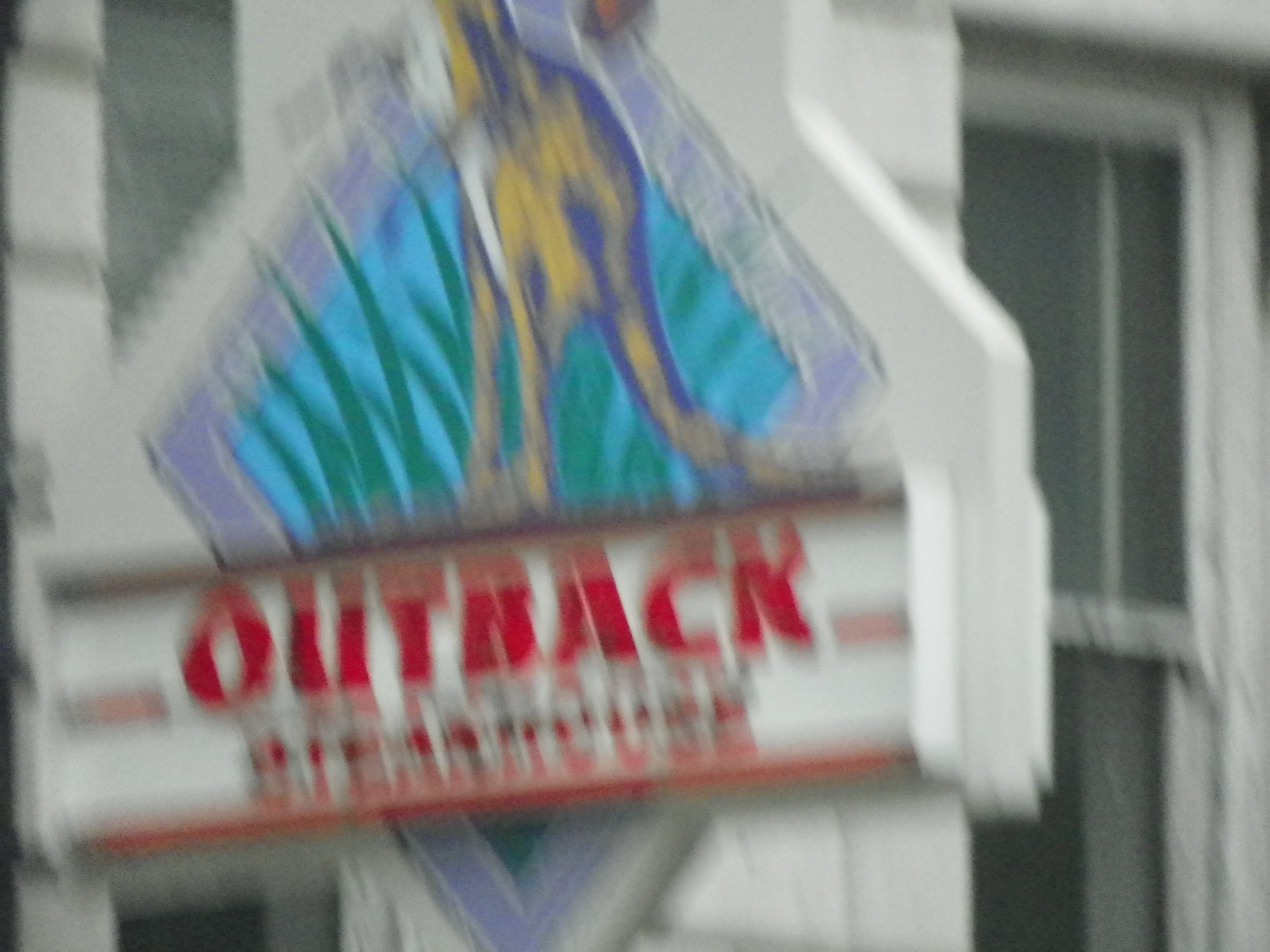This image is a very blurry photograph, presumably taken from a moving car, depicting the exterior of an Outback Steakhouse with its old logo. The sign prominently features the "Outback Steakhouse" name in large, red capital letters. This lettering is placed within a distinctive diamond-shaped border, which has a light blue outline filled with a sky-blue color. Surrounding the text are tall blades of dark green grass. Partially visible in the grass is a yellow illustration of a kangaroo, though the blur obscures the full animal, only showing part of its torso. The building in the background appears to be a residential structure, and the Outback Steakhouse's exterior seems to be made of light gray stone with a large dark window on the right side. The blurry quality makes it hard to discern finer details, but the overall composition captures the Outback logo amidst a somewhat suburban setting.